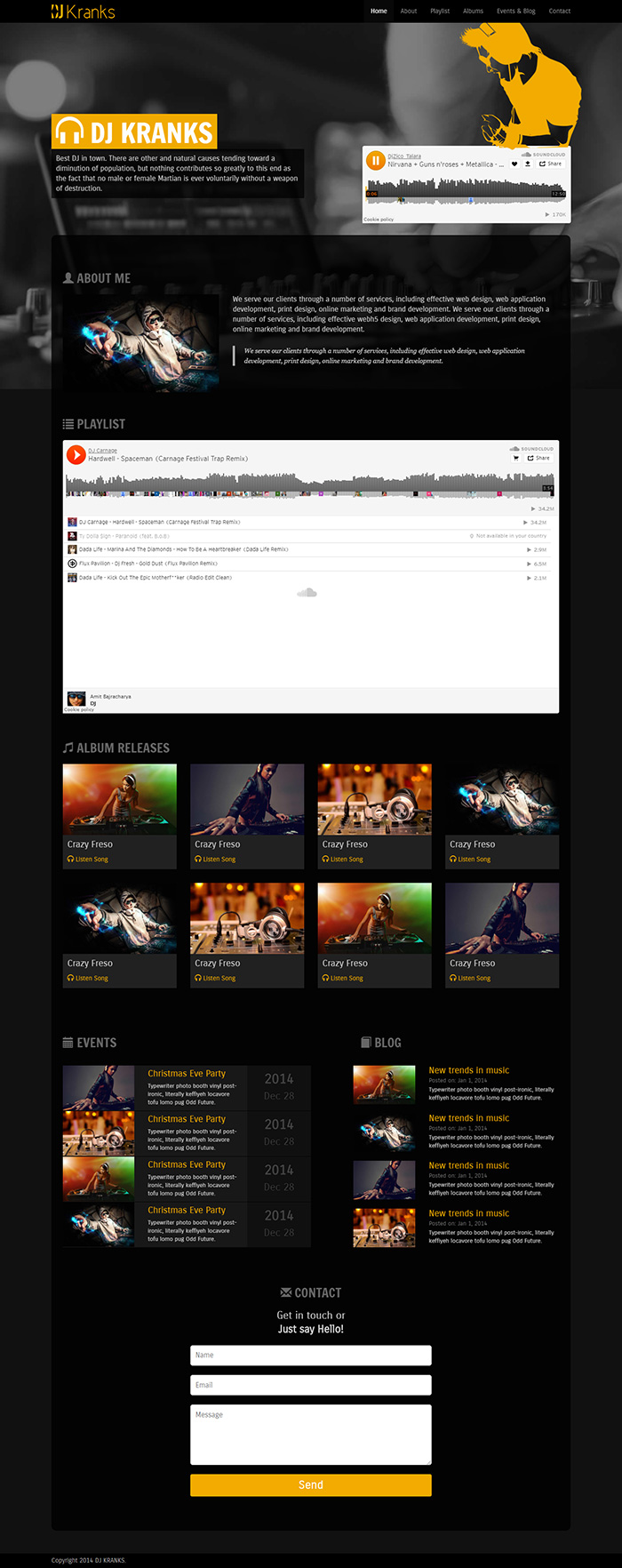This image is a screenshot of a mobile application featuring the artist DJ Kranks. The interface has a black background, offering a sleek and modern aesthetic. In the upper left-hand corner, a small, vibrant yellow rectangle prominently displays the text "DJ Kranks," suggesting the featured musician or artist of the application. To the right of this label, there is a segment showing a song currently playing, which could imply either a track by DJ Kranks or one affiliated with them.

At the bottom of the screen, there is a section showcasing eight albums attributed to DJ Kranks, allowing users to explore the artist's discography. Below the album list, there are details about events related to the artist, although the exact number is somewhat ambiguous—either four or eight events are listed. Lastly, the screenshot highlights four blogs written about DJ Kranks, providing additional context and insights into the artist's career and influence.

Overall, the image effectively highlights various aspects of DJ Kranks' presence within the app, including music, events, and media coverage, all neatly organized on a dark-themed interface for easy navigation and engagement.